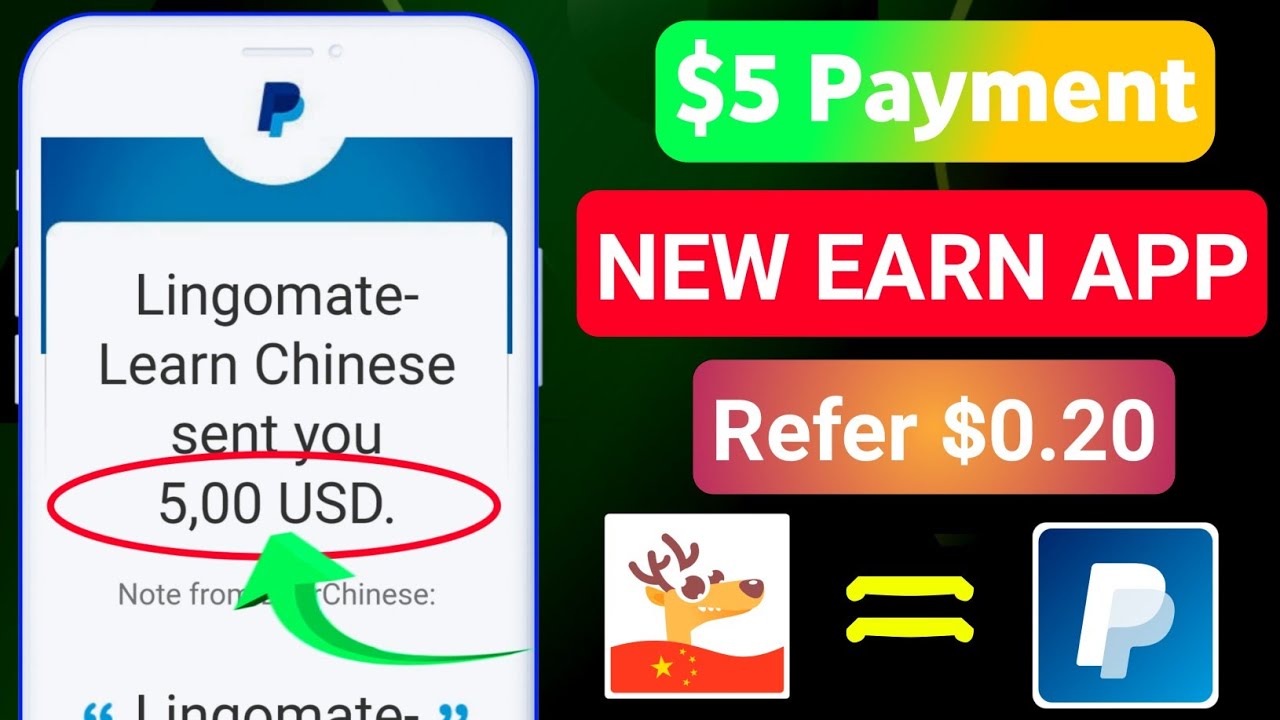The image features a black rectangular background. On the left side, there's half of a phone screen visible. To the right of the phone screen, occupying the remainder of the rectangular space, is a segment that displays the text "$5 payment" in white font. This segment has a gradient background transitioning from green on the left to yellowish-orange on the right.

Below this, there's another long rectangle with a red background that contains the text "New Earn App" in all capital letters and white font. 

Underneath, there's another rectangle that displays the text "Refer $0.20" in white. The background here fades from red to orange back to red.

On the phone screen to the left, at the top, there's a "P" logo, which represents PayPal. Below this logo, the text reads "Lingomate-LearnChinese sent you $5.00 USD."